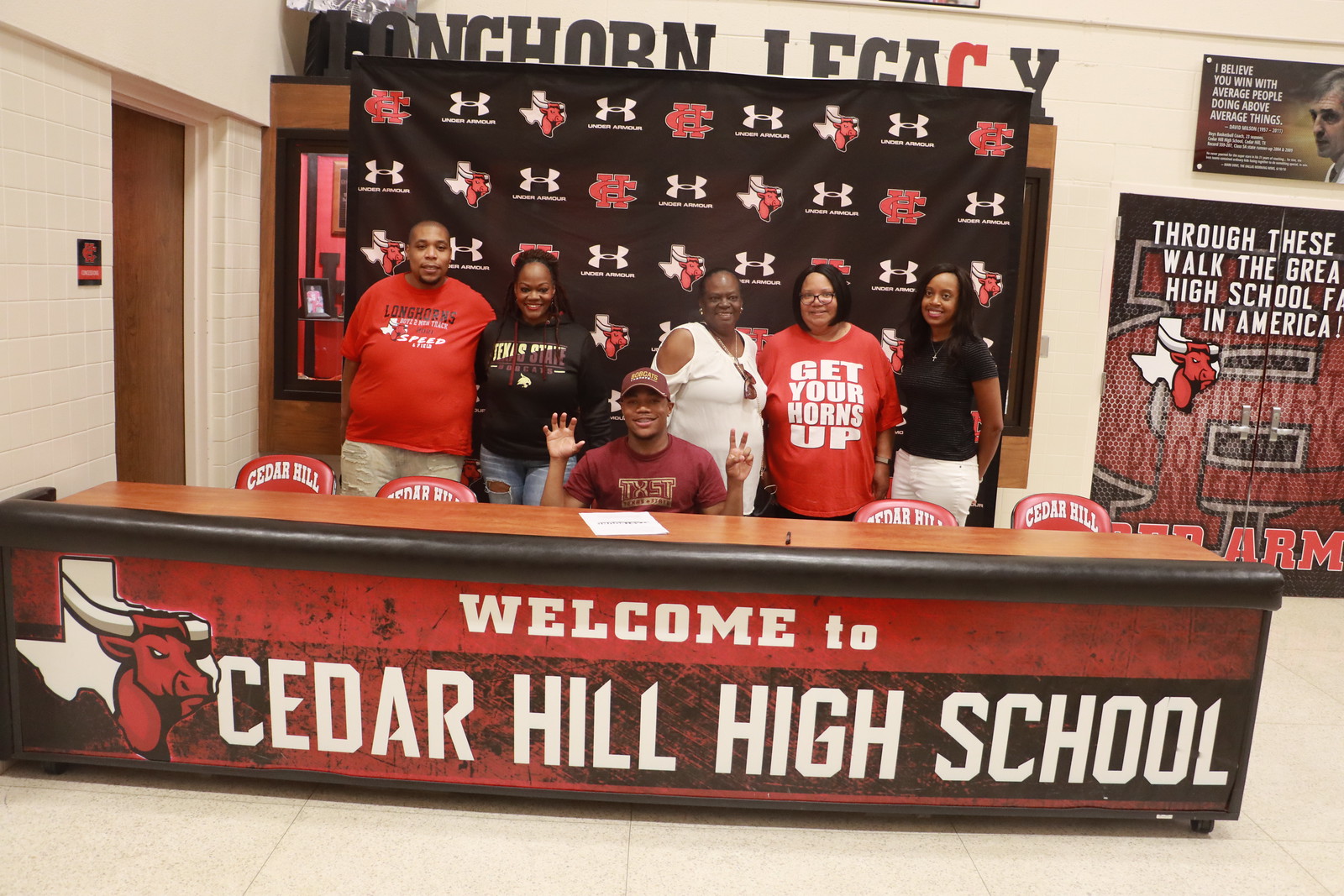This detailed horizontal rectangle image captured inside Cedar Hill High School prominently features a long bench with five chairs behind it. The bench’s front is inscribed with "Welcome to Cedar Hill High School" in large white letters, and above it sits a smaller welcome message alongside the school's logo - a stylized red bull with white horns superimposed on a partial silhouette of Texas. In the foreground, a man in a red shirt and hat holds his hands up, seemingly signaling the number 7, while seated at the bench. Surrounding him are four empty chairs.

Behind the bench, five individuals stand - one man and four women, dressed mainly in t-shirts of various colors, including red, black, and possibly dark red or purple. The backdrop comprises a black display, likely featuring alternating school logos and an Under Armour emblem, adorned with red elements. Above this display, the phrase "Longhorn Legacy" is visible, with "Legacy" emphasized in red. The wall behind them is white, contributing to the image’s overall color scheme of red, white, and black. This photograph seems to depict members of the Cedar Hill High School athletic department, possibly commemorating a significant event like a college sports signing.